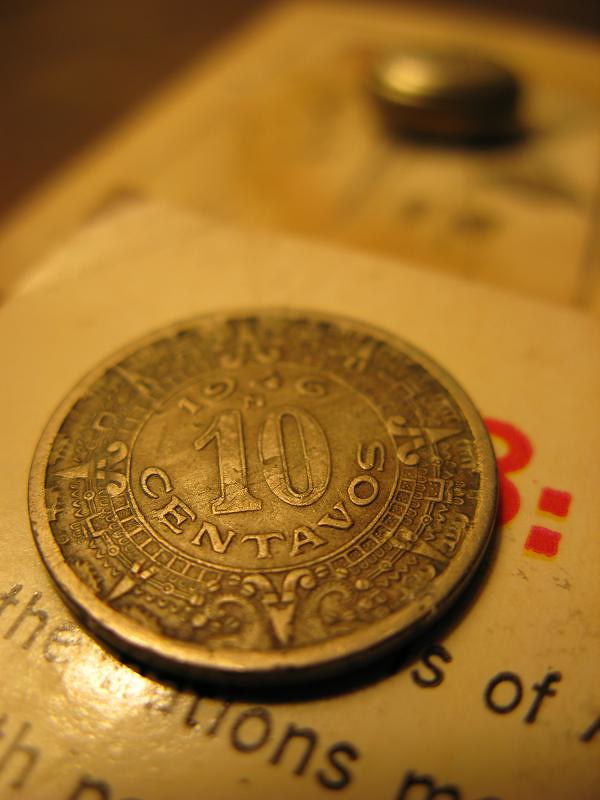This detailed image captures an extreme close-up of an aged, intricately decorated 10 centavos coin, prominently displaying the year 1946. The coin, featuring an elaborate sun-like design with intricate carvings around its circumference, is positioned face-up atop a tan, cardboard-like envelope. The background, largely blurred, adds to the photograph's focused depiction of the coin. The coin itself, silver with a tarnished bronze hue, is photographed at an angle, suggesting indoor settings due to the lighting and ceiling glare. Despite the surrounding blurriness, a metallic object can also be spotted on the tabletop.